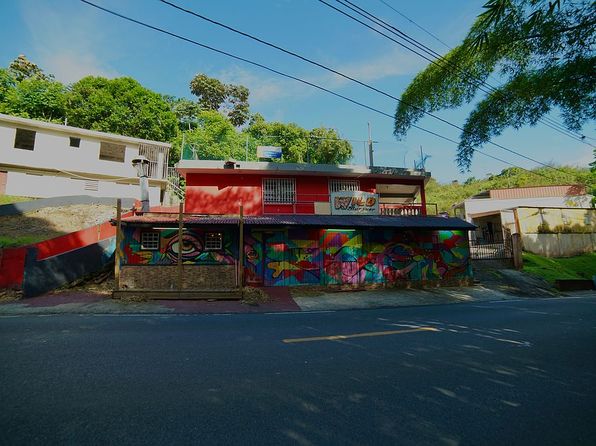This image portrays a vividly painted, two-story building along a paved asphalt road with a yellow stripe down the middle. The building, possibly a small restaurant or shop, is characterized by its eclectic and lively color scheme. The bottom story is divided into bright pink, green, and yellow sections, giving it an eye-catching appearance. On the left side, a small porch area is adorned with a large, brown eyeball mural flanked by two small windows. The awning above accentuates the boundary between the floors. The second level is dominated by a bright pink facade, featuring a poster with the letters "W-I-L-O," suggesting it might be related to a radio station, and includes a small balcony.

The building appears to be in a somewhat rundown or economically challenged area, with a "shacky-ish" look and a slightly slanted roof. Surrounding elements include a concrete sidewalk, a street with an incline, power lines draped over the buildings, and trees visible in the background. A fence can also be spotted, adding to the scene's eclectic urban landscape. Overall, the building stands out dramatically against its more subdued surroundings, primarily due to its vibrant and artistic exterior.